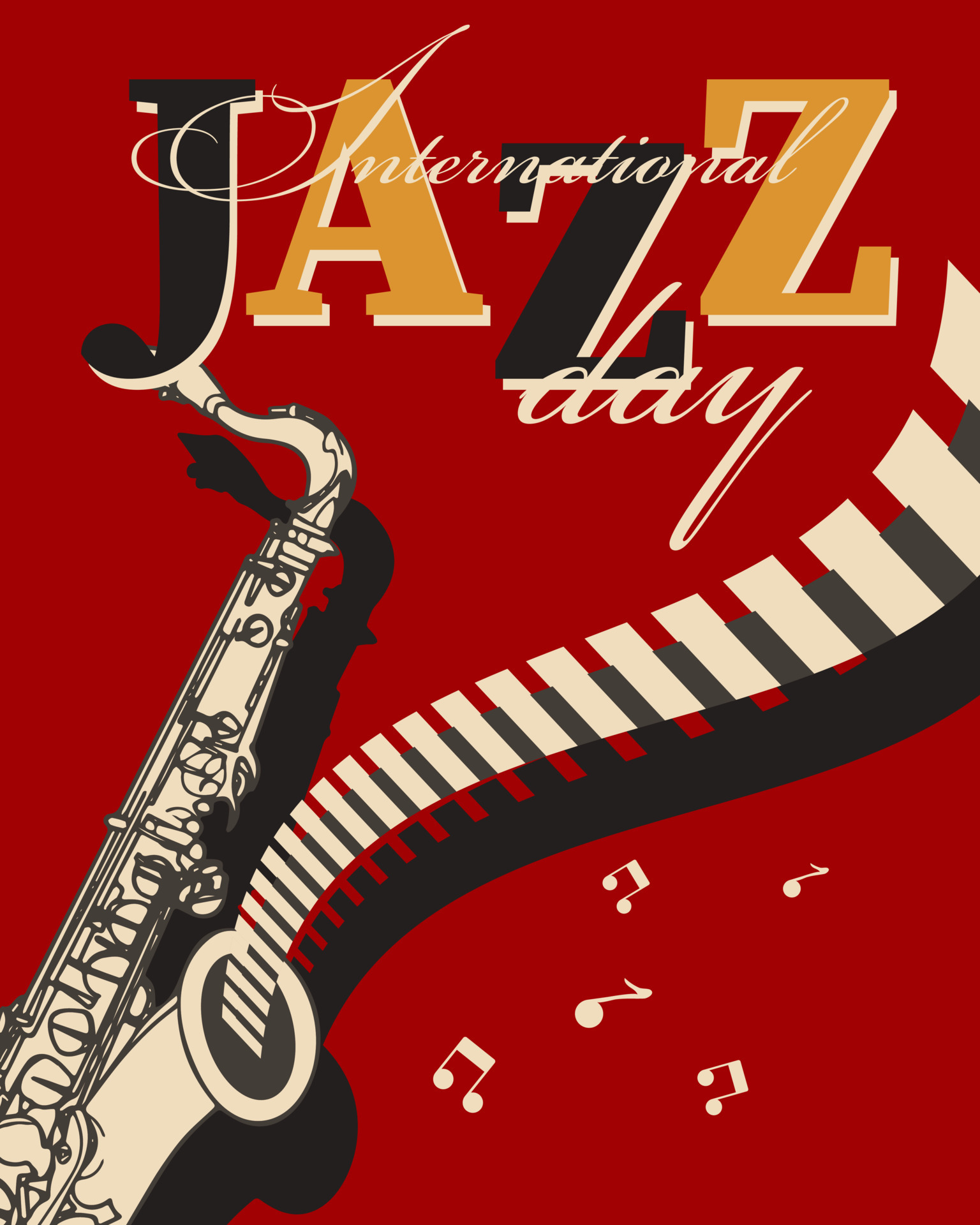This is a graphic-designed poster for International Jazz Day set against a deep red background. At the top, the word "JAZZ" is prominently displayed in large, playful block letters; the J and first Z are black with white shadows while the A and second Z are golden with white shadows. The letters are arranged in a dynamic layout, giving a sense of movement. Superimposed across these letters in delicate white cursive font are the words "International Day." Below the text, a cream-colored saxophone illustrated with black details is central to the design. Emerging from the saxophone is a creative depiction of musical notes resembling piano keys, accompanied by additional white music notes scattered throughout the image, adding a lively and harmonious touch. The saxophone and musical elements cast a dark black drop shadow, giving depth to the poster.